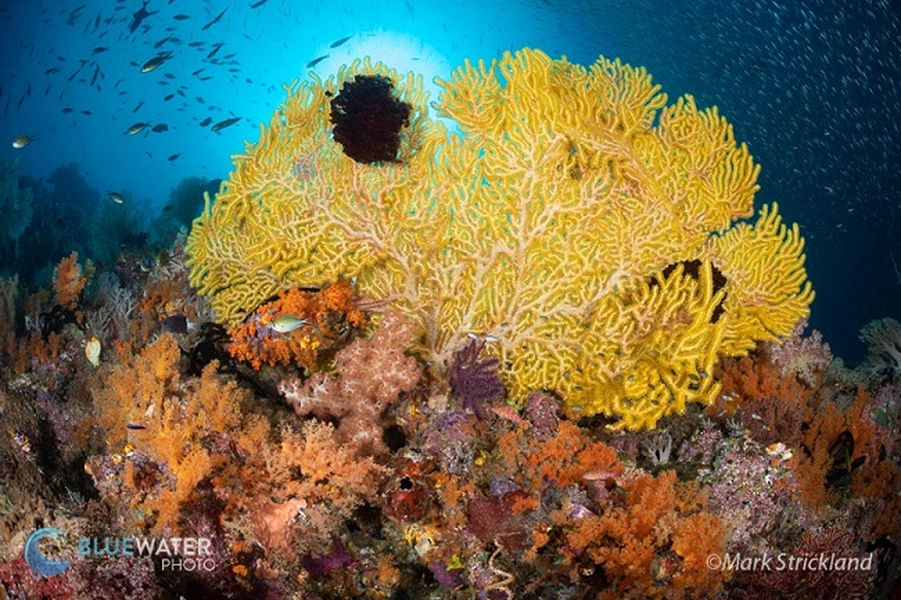The underwater scene is teeming with vibrant plant life, indicative of a reef or a shallow water area. A diverse array of organic material and fish populate the image, creating a lively and colorful ecosystem. Prominently featured are pink and red hues, possibly coral, alongside striking orange tones. Central to the composition is a large, yellow coral structure resembling a tree. The seabed also features shades of brown and darker colors, suggesting a rich, varied environment. Within the yellow coral structure, two very dark circles are visible, potentially small schools of black fish. Numerous fish of varying sizes and colors, both light and dark, swim around this focal point. The entire scene is bathed in light filtering through the blue water, illuminating the distant aquatic life and adding depth to this underwater tableau.